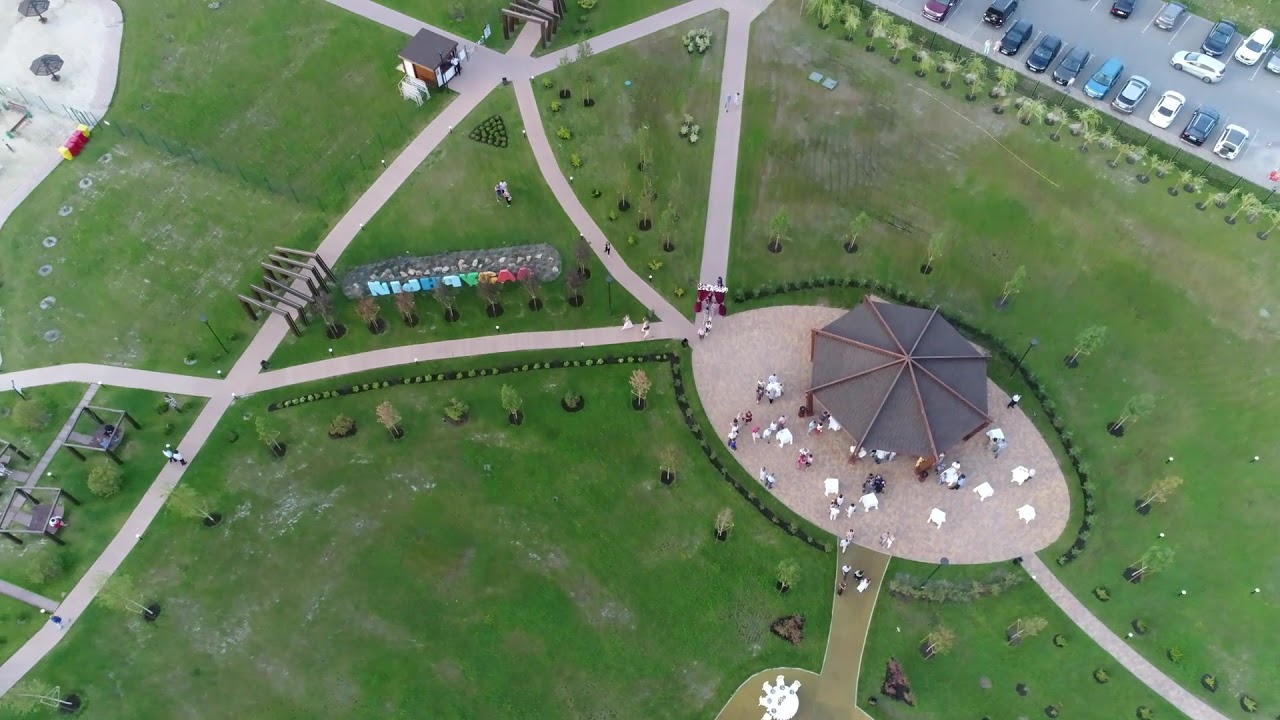This aerial photograph captures a sprawling, lush green park interwoven with light cream-colored pathways. These pathways diverge and converge throughout the garden, leading towards and originating from a central, oval-shaped area. In this focal area, there's a large, gray-colored umbrella standing prominently amidst white chairs and people who are mingling. The pathways and the central area share the same cream tone, creating a harmonious look. Alongside the pathways, various trees and bushes are planted, forming a picturesque network of greenery.

In the upper right-hand corner, just beyond the bounds of the garden, a parking lot fills with neat rows of vehicles separated by white lines. Adjacent to this, a row of small sapling trees provides a natural buffer. The park also features several distinct sections, including a paved area in the upper left with playground equipment and a stone wall adorned with colored lettering in a rainbow pattern. Just left of this wall, a short covered passage framed by brown door frames leads to another area, marked by a small building and enclosed with a fence, indicating an entrance to a restricted space. This detailed layout of the park encapsulates the serene beauty and intricate design of the recreational space.